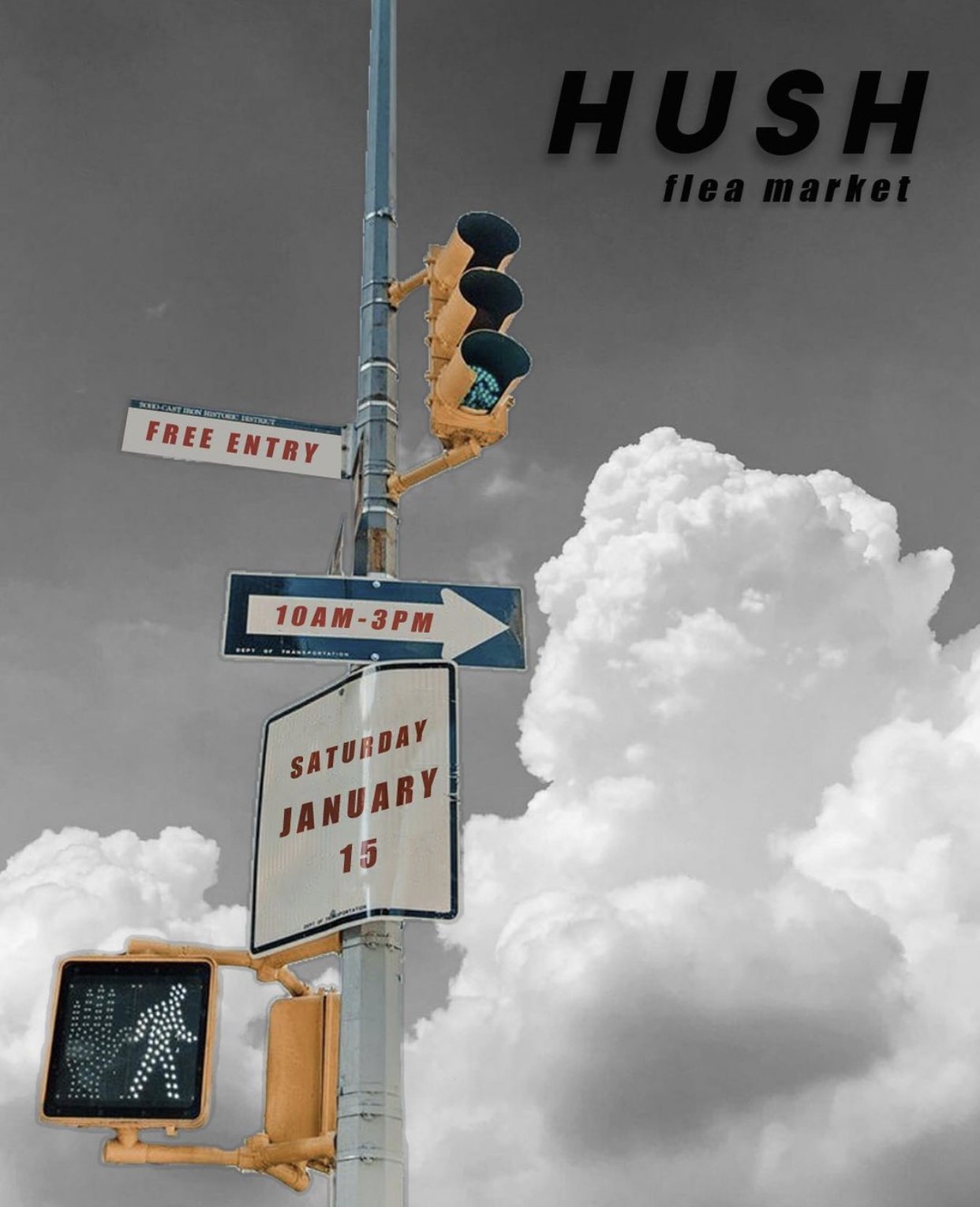The image captures a scene against a gray sky backdrop with prominent white clouds. In the top right corner, black text reads “HUSH FLEA MARKET.” Towards the middle-left side of the image, a silver traffic light pole stands, featuring a green-lit traffic light with a yellow casing. Below the traffic light, a series of signs are attached to the pole. The uppermost sign, bordered in red on a white background, announces “FREE ENTRY.” Directly beneath it, a black sign with a white arrow pointing right displays the time “10 AM to 3 PM” in red text. Below this, another sign with a black outline and white background lists the event date: “SATURDAY, JANUARY 15TH.” Finally, at the base of the pole, a pedestrian signal shows a lit walk symbol, indicating a safe crossing time. Whitesmoke is visible billowing from the bottom left and right edges of the image, adding to the atmospheric scene.